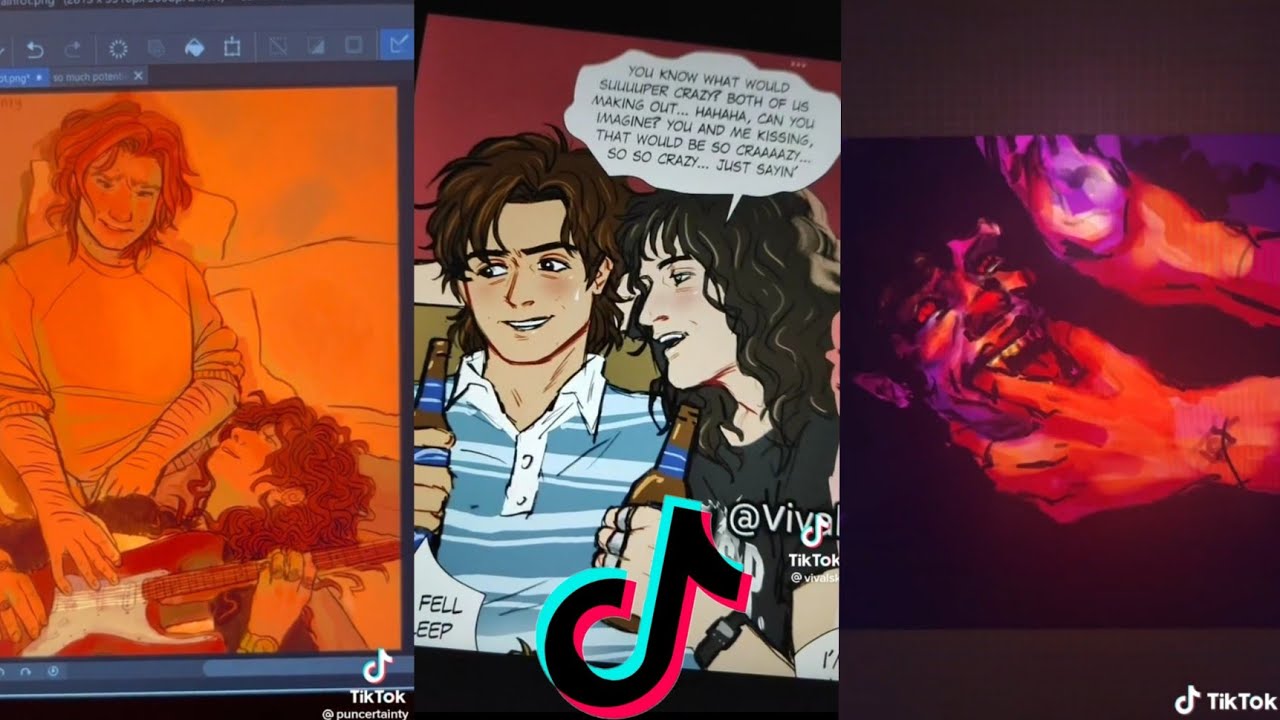A screenshot from a TikTok post, presented in three graphic panels. The first panel, set against an orange sepia overtone background, depicts two male friends in a cozy scene. One friend, with reddish hair, is playing a guitar, while the other, sitting beside him and also interacting with the guitar, strums the strings. The intimate moment captures their shared musical bond. 

In the second panel, the vibrant orange tones disappear as the scene becomes more realistic. The friend on the right, sporting shaggy brown hair and clad in a blue and white striped polo shirt, converses with the friend on the left, who has long curly brown hair and wears a black T-shirt. A speech balloon from the friend in the black T-shirt reads humorously, "You know what would be super crazy? Both of us making out, ha ha, can you imagine? You and me kissing, that would be so crazy. So, so crazy, just saying." A TikTok watermark at the bottom confirms the post's origin.

The third and final panel shifts dramatically in tone, featuring what appears to be two hands reaching towards a distorted, vampiric face. The dark, eerie face amalgamates purple and red overtones, offering a spooky contrast to the previous lighthearted interactions.